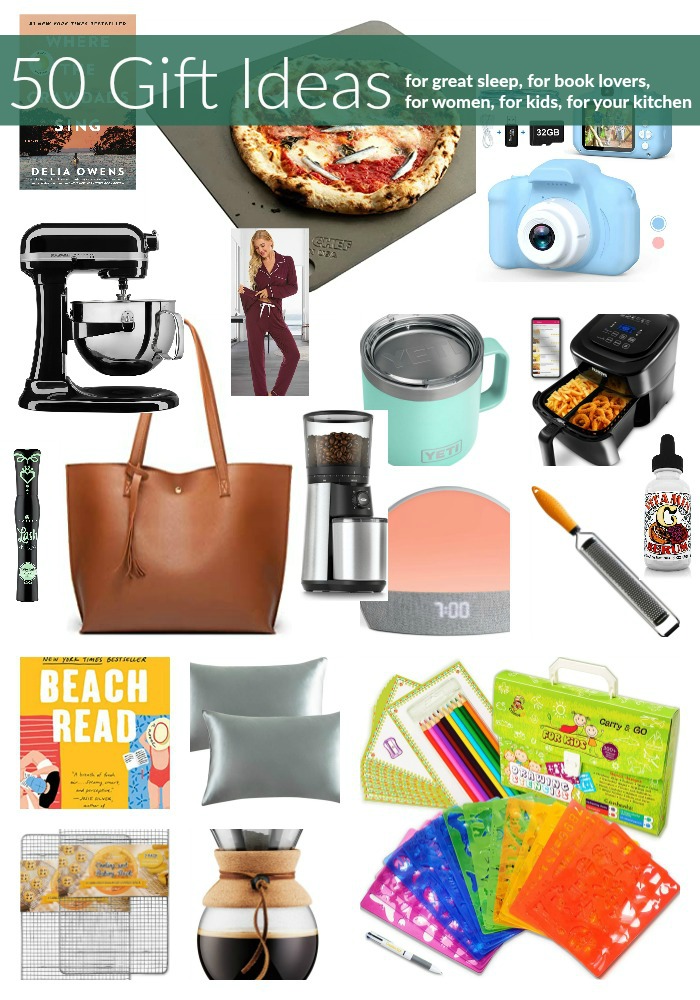This image is a detailed collage of various gift ideas, likely featured on an e-commerce website, designed to cater to a variety of interests such as great sleep, book lovers, women, kids, and kitchen enthusiasts. At the top of the image, there's a prominent green banner with bold white text stating "50 Gift Ideas." To the right of this text, in smaller font, are the categories: "for great sleep," "for book lovers," "for women," "for kids," and "for your kitchen."

The array of items included as gift suggestions are strategically placed on a white background. Key items in this collage include:

- A green KitchenAid mixer.
- A model wearing wine-colored pajamas.
- A baby blue Polaroid digital camera.
- A sturdy Yeti mug.
- An air fryer.
- A coffee grinder.
- A brown pocketbook.
- A book titled "Beach Read."
- Silver satin pillows.
- A children's carry-and-go stencil drawing set.
- A shiny black espresso machine.
- A simplified alarm clock indicating seven o'clock.
- A slice of pizza on a stone platter.
- Various other utensils like a grater for zesting citrus and a wireframe grilling sheet.
- A glass coffee pot wrapped in a cozy.
- A wake-up light alarm clock.

In addition, there are obscure items like a black tube featuring a Native American face, making the collection visually diverse and intriguing. This arrangement aims to offer visually appealing examples from the broader list of "50 Gift Ideas," capturing attention with its vibrant mix of items for different consumer needs and interests.